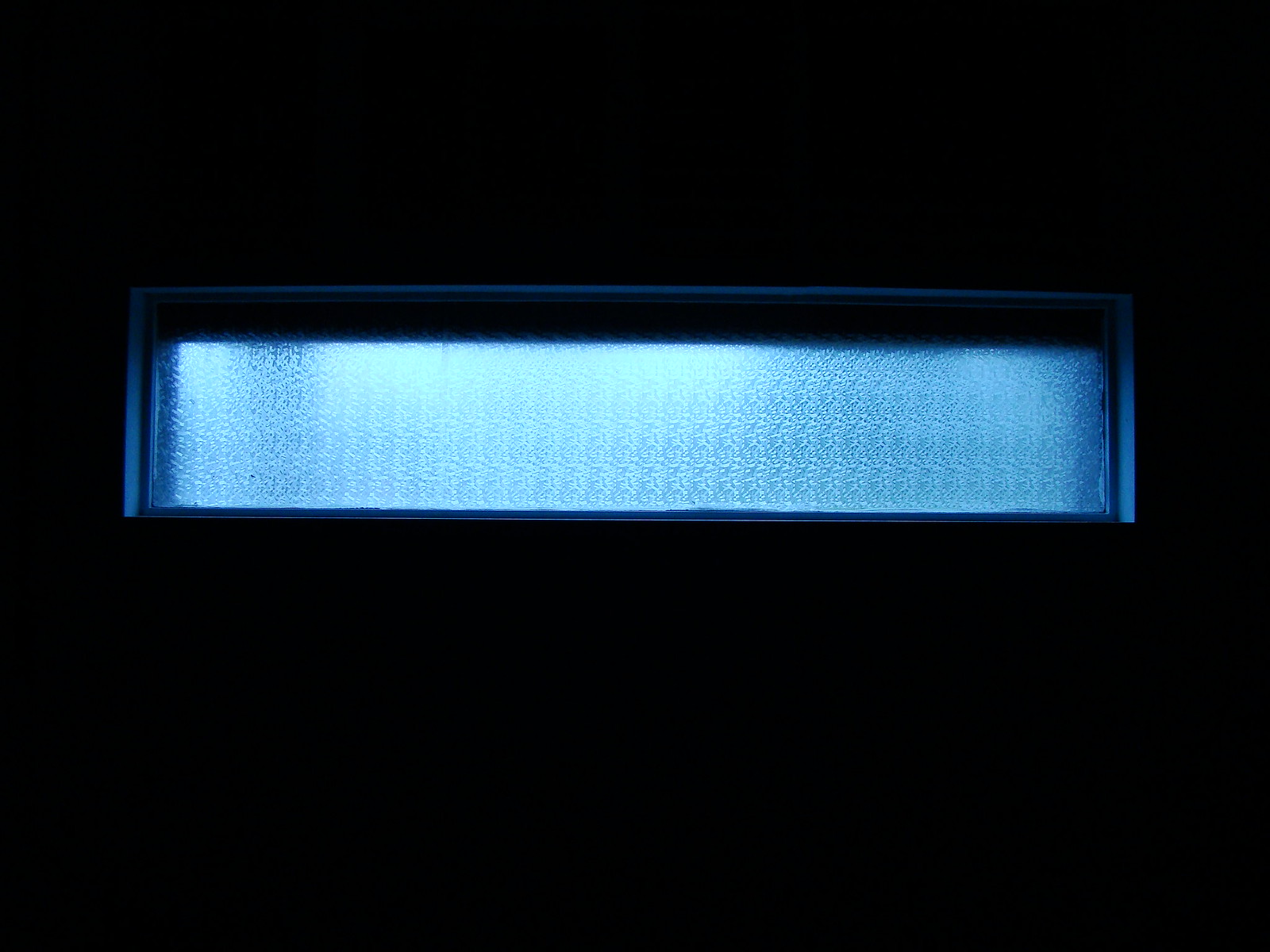This photograph features a predominantly pitch-black background, highlighting a single, central element: a horizontal, rectangular bar with a silvery blue hue. Positioned slightly in the upper half of the image, this bar has a textured, almost fabric-like appearance that suggests a smooth material. The light reflecting on it reveals varied shades of blue due to the angle and intensity of the illumination, which appears to come from a bit left of center and slightly above.

The bar is encased in a matching blue outline, giving it a framed look that resembles a sunken element in an otherwise completely dark wall. Only the topmost part of this bar immerses into shadow, nearly blending into the pitch-black background but leaving the distinct outline visible. The resulting visual effect makes it unclear whether this is a piece of art, a frosted window, or another form of illuminated installation. This ambiguity, combined with the stark contrast of the illuminated bar against the pure black background, makes for a striking and mysterious composition.